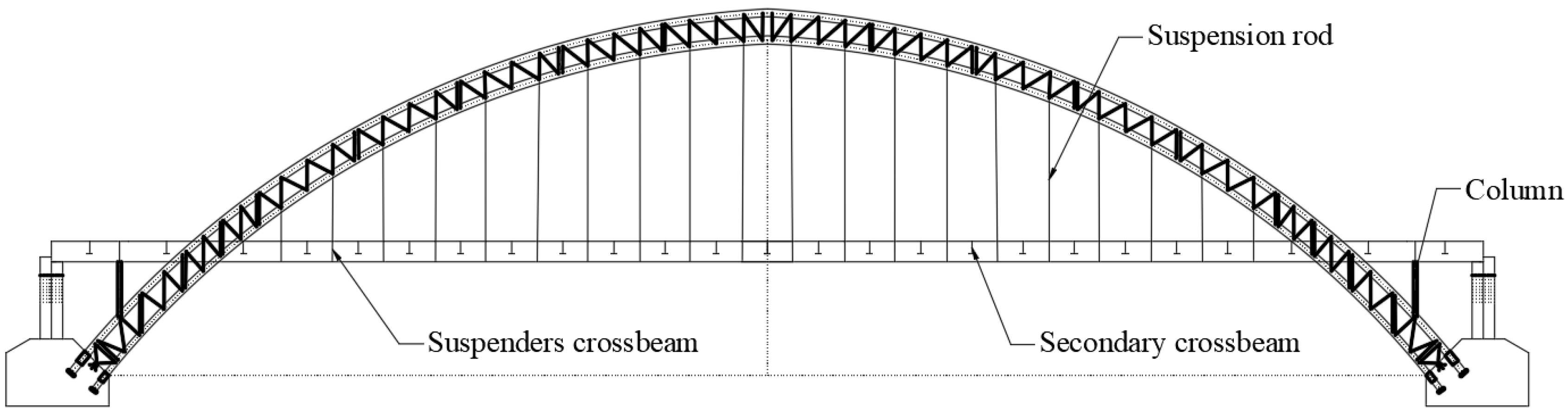The image is a detailed black-and-white architectural schematic of a traditional bridge, reminiscent of the San Francisco Bay Bridge. This rectangular diagram with a white background features a prominent beamed arch over the bridge deck. Connecting the arch to the flat horizontal surface of the bridge are numerous vertical suspension rods. These rods extend downward through a small space before connecting to another structural element labeled as the suspenders cross beam.

Additionally, nestled between the suspension rods at the bottom section are vertical hash marks that denote the secondary cross beam, which doesn't reach entirely to the bottom of the section. On both ends of the arched structure are heavy black lines labeled as columns, which span from the top of the arch down to what looks like large stone or cement bases that anchor and stabilize the entire bridge. The schematic includes annotations pointing out key structural components such as the column, suspension rod, secondary cross beam, and suspenders cross beam, highlighting the fundamental design of a traditional yet robust bridge structure.